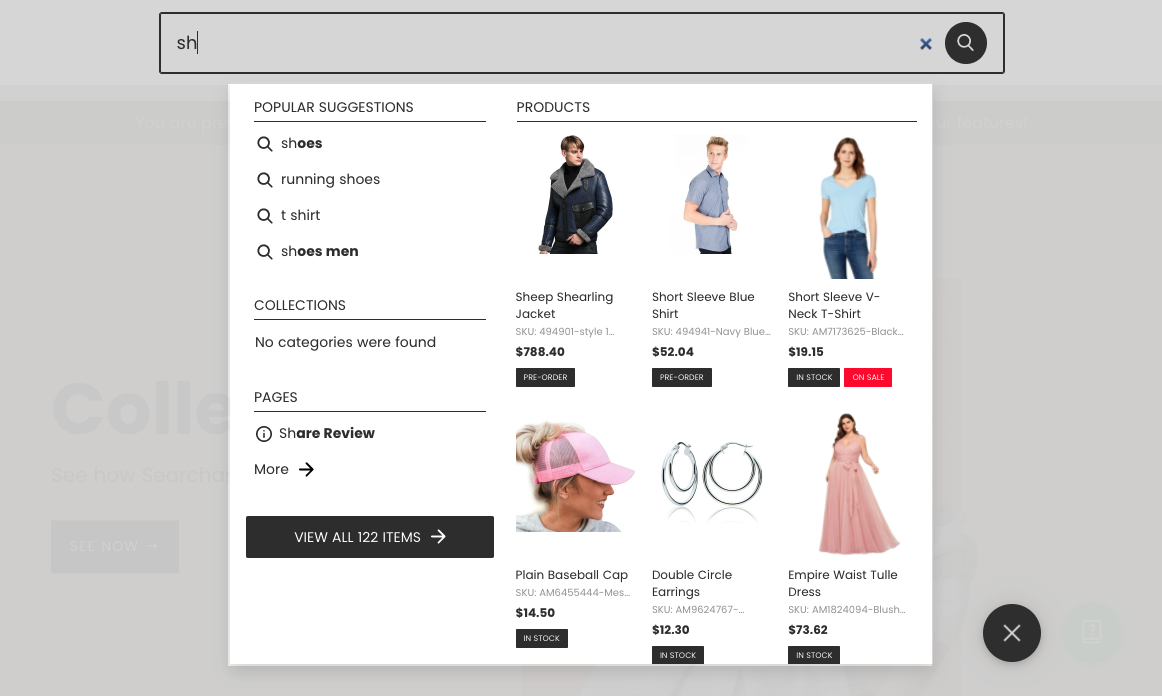This screenshot captures the search results from an online clothing and accessories retailer. The search query "SH" yields popular suggestions including "shoes," "running shoes," "t-shirt," and "shoes men." The results are filtered under collections, although no specific categories were found. The user can view all 122 items, but only six products are currently visible in this image:

1. A luxurious Sheep Shearling Jacket priced at $788.40.
2. A Short Sleeve Blue Shirt available for $52.04.
3. A Women's Short Sleeve V-neck T-shirt costing $19.15.
4. A Plain Pink Baseball Cap priced at $14.50.
5. A pair of Silver Double Circle Earrings listed for $12.30.
6. A Pink Empire Waist Tulle Dress, a long gown, priced at $73.62.

Above the product listings, navigation options include "collections," "share review," and links to various store pages. This assortment showcases a variety of styles and price points, offering a comprehensive snapshot of the store's diverse inventory.